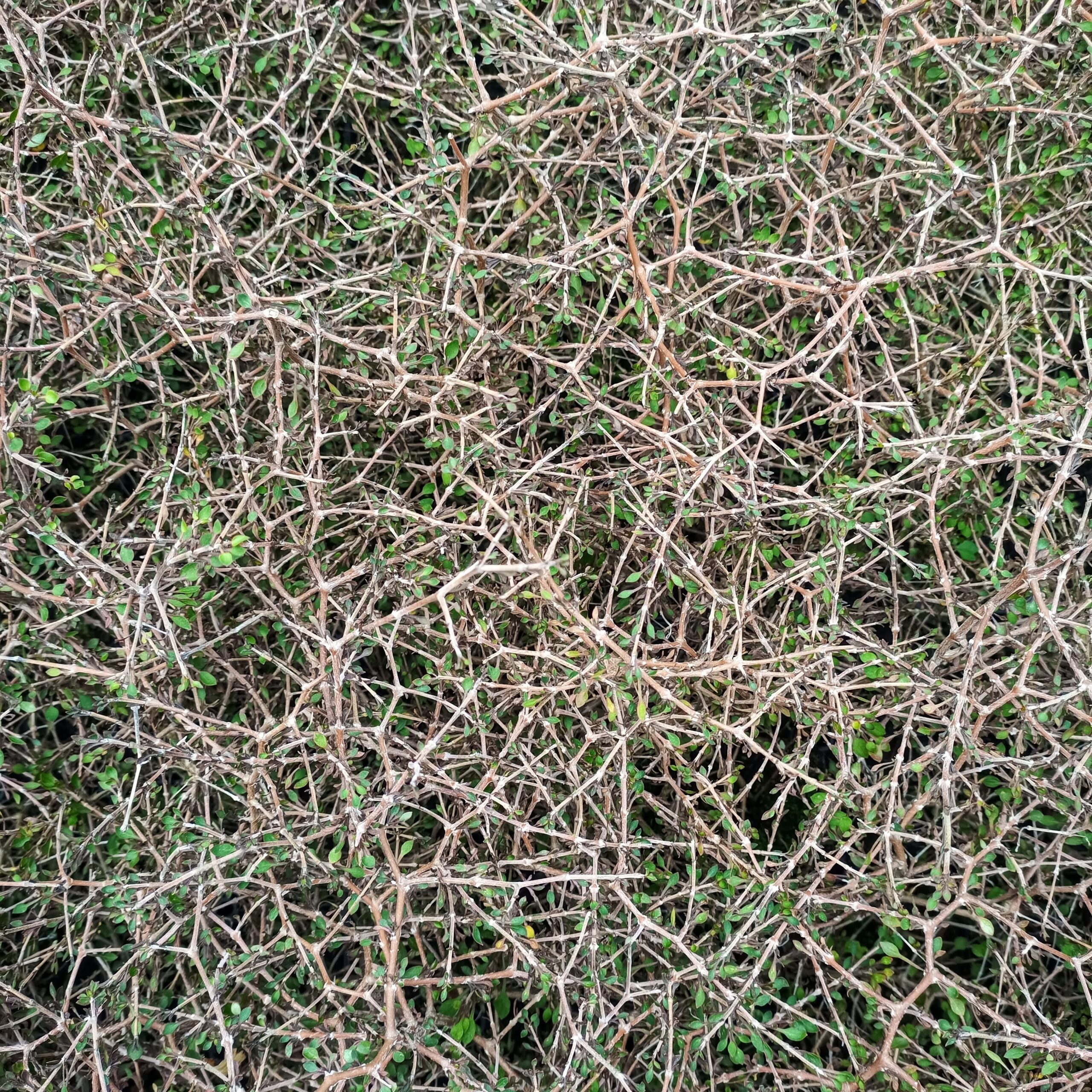The photograph depicts a detailed, top-down view of a dense ground cover composed primarily of thorny Vela Spinosa plants, also known as the crown of thorns and native to Spain. The entire frame is a tapestry of interwoven light brown and gray twigs that form a crisscross mesh resembling a natural web, creating a complex and unique texture. Beneath this intricate layer of twigs, small green leaves and patches of weed grass peek through, contrasting against the dark earth beneath. The image, consistent throughout, highlights the intricate, tightly woven pattern of the Vela Spinosa's thorny structure, punctuated by the occasional green sprout, offering a fascinating texture that could serve as a background or illustrative detail.